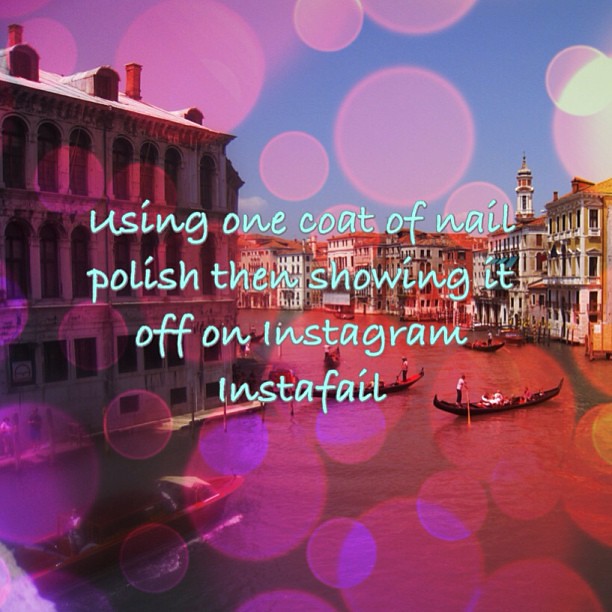The image is a humorous, Instagram-style post featuring a picturesque cityscape that resembles a blend of Venice and Shanghai, characterized by old European-style buildings with numerous windows, some reaching three stories high. In the foreground, a serene river is traversed by four to five rowboats, possibly operable for hire, giving the impression of a bustling, scenic area. The entire scene is overlaid with a pinkish filter, accented by subtle, bubble-like circles, creating a whimsical aesthetic. Centered in the image is a playful text in stylish blue font that reads, "Using one coat of nail polish, then showing it off on Instagram, insta-fail," adding a humorous twist to the scenic background.